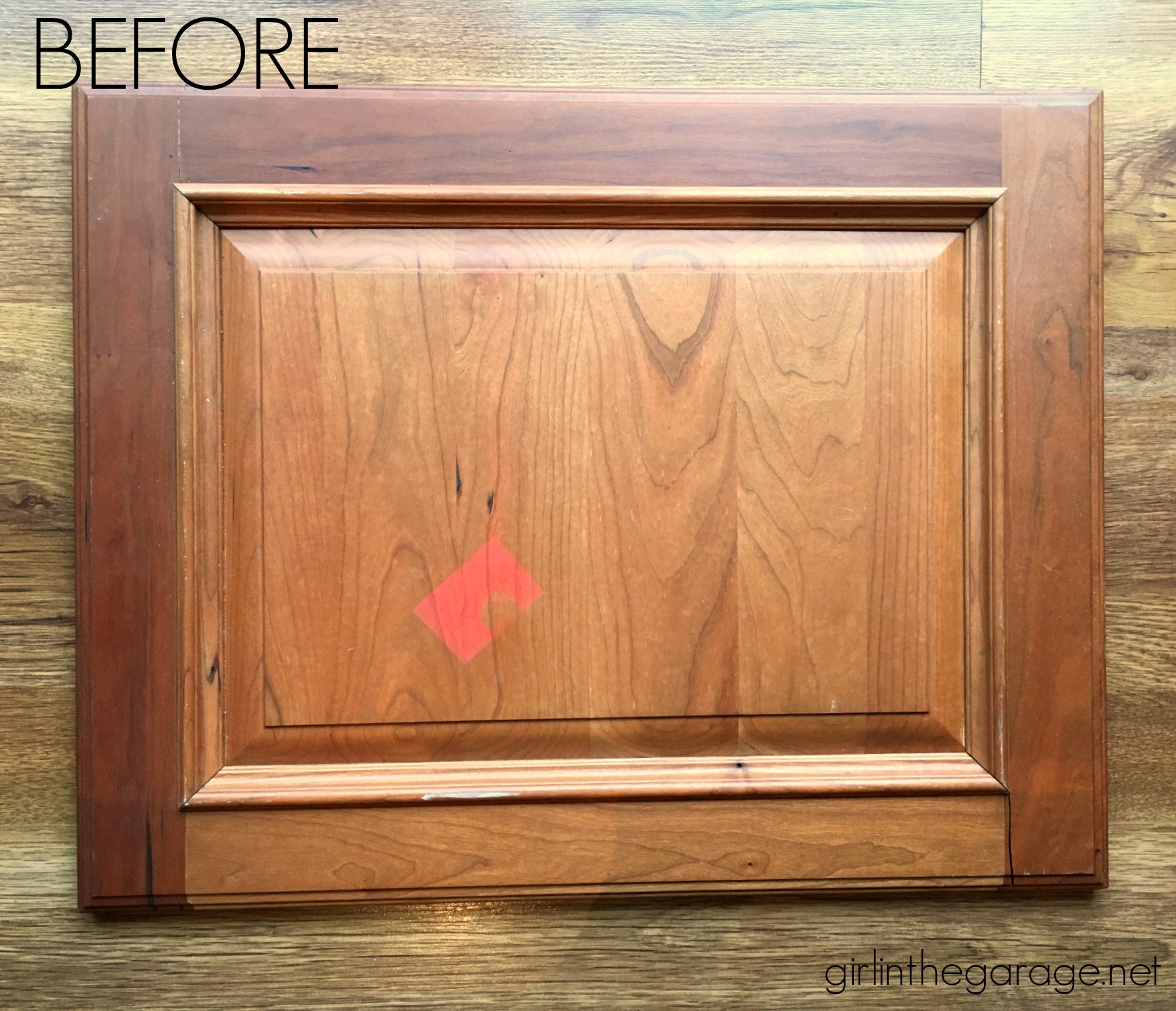The image depicts a cabinet door panel, likely destined for a kitchen, positioned on a dark hardwood floor. The door, which appears to be made from a mix of hardwoods, perhaps oak, showcases a rich, deep coloring with lighter tan hues. It features molding around the edges and displays wood grain indicative of its material. Notably, there is a diagonally placed, partially removed red sticker or square, suggesting some residue or stickiness on its surface, possibly indicating the need for restoration. The image includes text: "BEFORE" in black letters in the top left corner, and "girlinthegarage.net" in black letters in the bottom right corner, emphasizing that this is a 'before' picture of a restoration project.